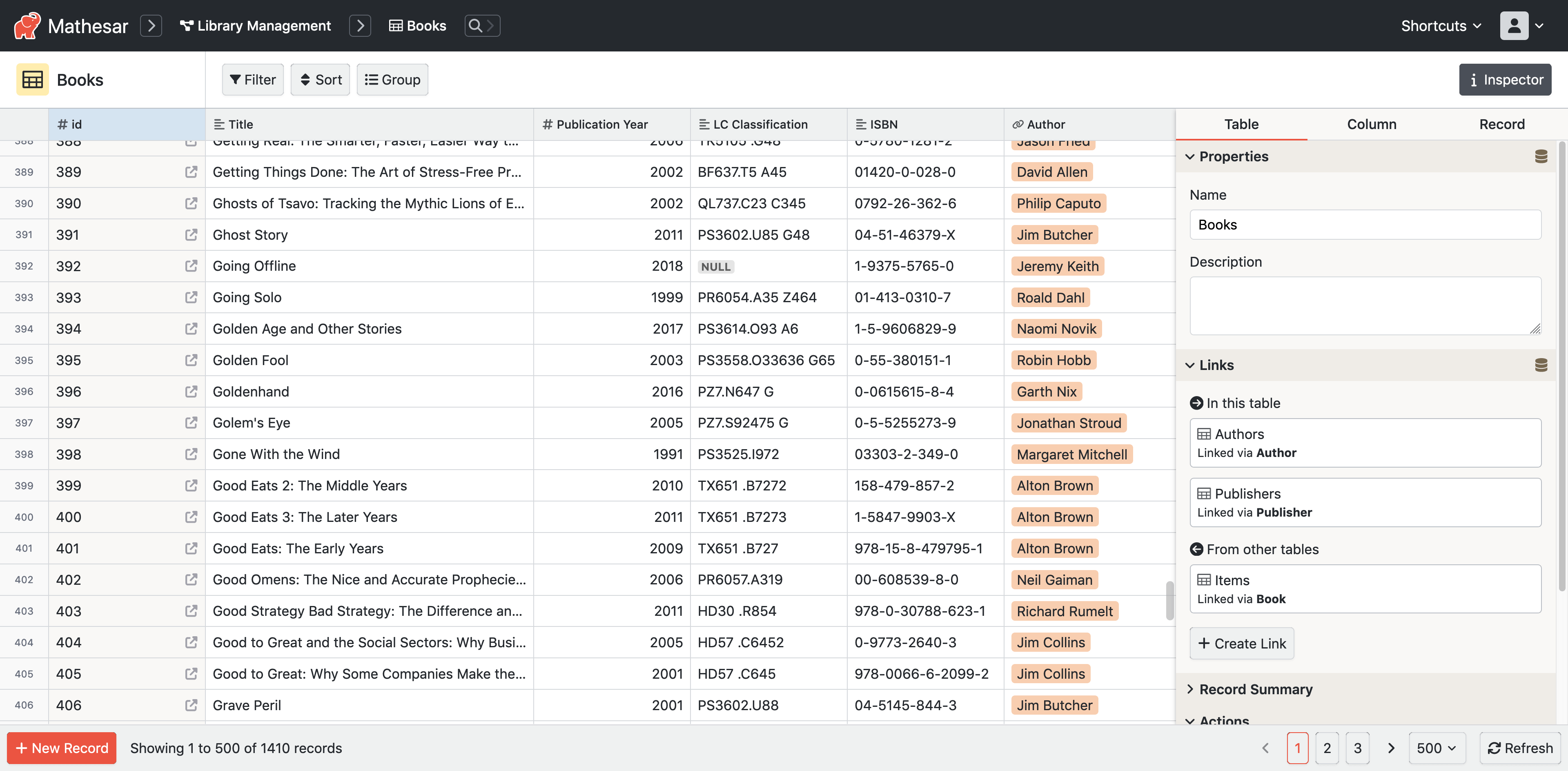This image showcases a webpage from a library management system known as "Mathis R." In the upper left-hand corner, the title "Library Management" is prominently displayed, serving as a header for the page. The interface is primarily white with black letters and features a black horizontal bar running across the top, providing a clean and structured layout.

The webpage is organized in columns resembling an Excel spreadsheet. The first column is labeled "Number ID," listing identification numbers starting from 388 at the top and going down to 406 at the bottom, arranged in alphabetical order. For instance, entry number 389 is titled "Getting Things Done: The Art of Stress-Free Productivity," while entry number 395 is "Golden Fool." Entry number 400 is titled "Good Eats Three: The Later Years," and entry number 405 is "Good to Great: Why Some Companies Make the Leap...and Others Don't."

The next column outlines the publication year, which ranges from 1991 to 2018. This column is followed by a "Classification" column that includes identifiers like "TX651.87272," and an ISSN number such as "158-479-872-2." Further details include the names of the authors, with examples like Robert Ronald Dow, Alton Brown, and Neal Gaiman listed.

Additionally, there is a "Shortcuts" section located to the right of the screen, providing quick access to various functionalities of the library management system. The far right-hand column offers search options, detailing the book names, descriptions, and links for further navigation.

At the bottom of the screen, pagination controls allow users to flip through multiple pages of the library catalog, further enhancing usability. This screenshot effectively captures the structured and comprehensive layout of a library management webpage, designed for efficient navigation and detailed book listing.